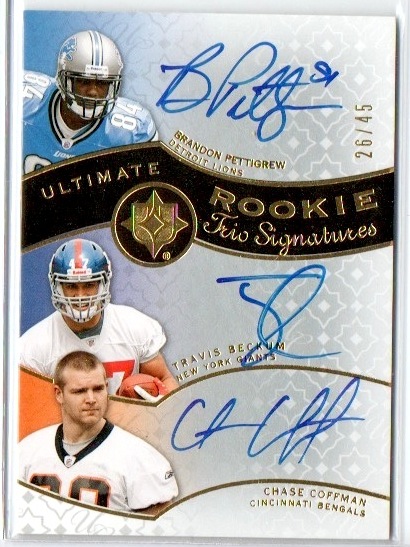This image showcases a highly detailed, autographed football collector's edition card titled "Ultimate Rookie Trio Signatures." The card features a white background adorned with a flowery design on the right side and a black strip with a golden band running vertically down the middle. The top section highlights Brandon Pettigrew of the Detroit Lions, with his picture on the left in a blue uniform with a silver helmet. Above his image is his blue signature. Below this, in gold print on the black strip, it says "Ultimate Rookie Trio Signatures." 

In the midsection, the card features Travis Beckham of the New York Giants. His signature is also in blue ink, positioned above his image on the left, where he is seen holding a football in a red and white uniform with a blue and red helmet. 

At the bottom, Chase Kaufman of the Cincinnati Bengals is depicted in his white, orange, and black uniform, standing helmetless. His blue signature is positioned above his photograph. The card also features an inscription rotated 90 degrees counterclockwise on the right side, marking it as "26/45" in gold text.